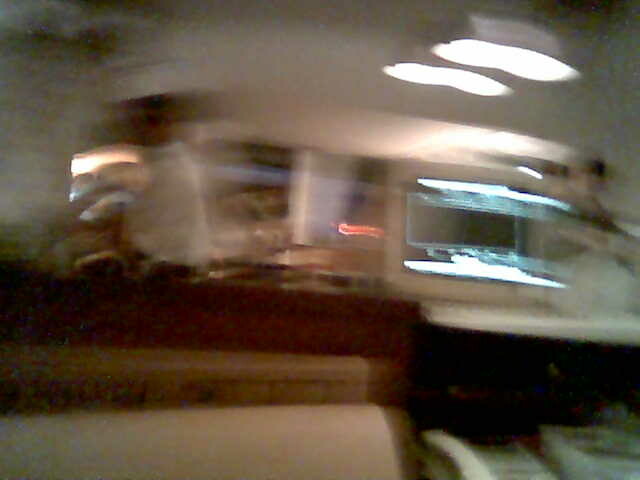This blurry and out-of-focus image appears to be taken inside a restaurant, likely an older-style establishment with booths and high wooden backs. In the lower left corner, part of a white booth seat is visible. To the left center of the photo, there's a male figure in a white long-sleeve shirt and black pants who might be either walking or engaged in some activity. His presence is somewhat obscured by the blurriness. The right side of the image shows a white table or counter against a black floor. In the background, through a window, various colored lights—blue, red, and others—can be seen. At the very top right of the picture, bright ceiling lights illuminate the scene. There might also be a TV or another fixture mounted on the wall near the center right, but the lack of focus makes it indistinguishable. Overall, the photo captures a bustling, yet indistinct moment in what seems to be a diner or casual restaurant.